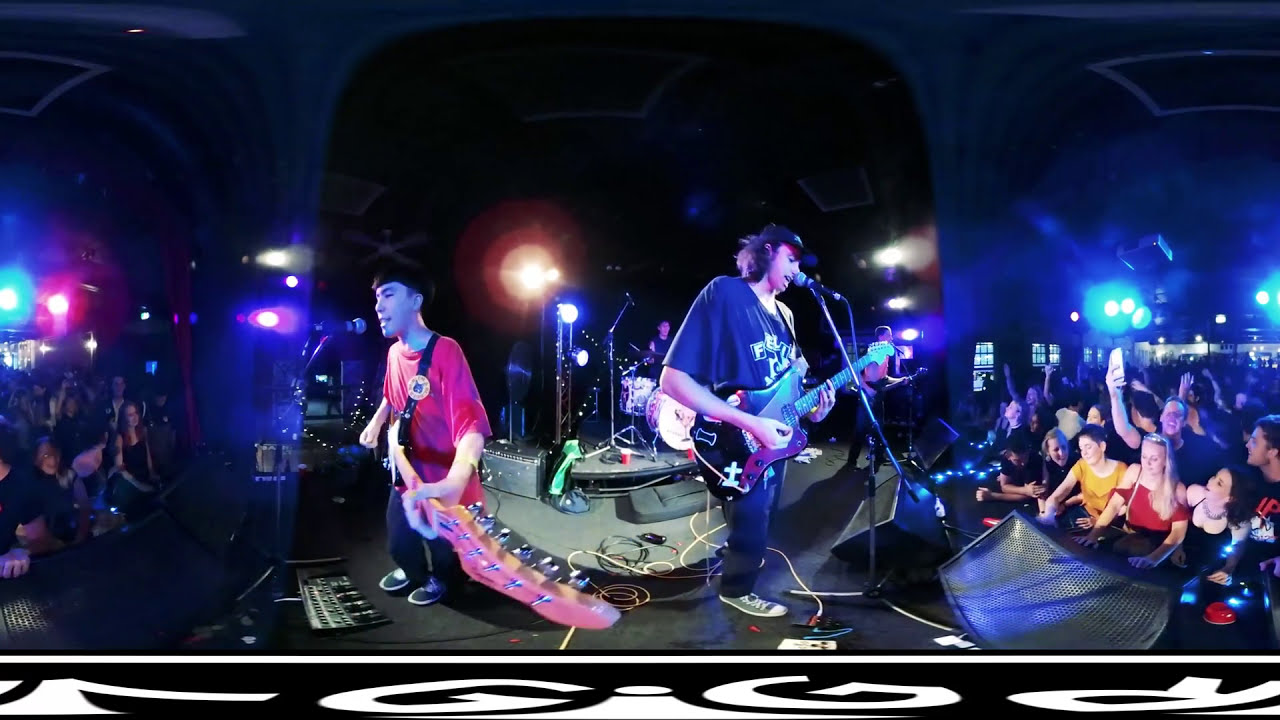In this concert image, the scene is bustling with energy. Central to the photograph is the stage, where three musicians captivate the audience. The guitarist on the right wears a black shirt and black pants, complemented by gray Converse shoes. He’s singing into a microphone with a baseball cap covering his long black hair. On his left, a musician in a red shirt and black pants plays a pink, somewhat distorted electric guitar due to the photo's curvature. There's also a drummer positioned behind them, set up slightly elevated.

To the right of the stage, you can see several concertgoers standing at a bar and engaging in conversations. Among them is a woman in a black top, another in red, and one in yellow. Most of them have their hands resting on the countertop, their attention partially divided between their drinks and the performance. Behind the bar group, a man is captured taking a selfie. Further back, some dimly lit windows contribute to the atmospheric setting, creating shadows in the upper right corner of the image.

On both sides of the image, the audience extends outward, enveloping the stage in a way that suggests this might be a stitched 360-degree view. The stage and the instruments appear somewhat warped and curved, enhancing the immersive feeling. Brightly colored lights—blue and red—illuminate the venue, highlighting the concert’s nighttime ambiance with an array of hues, including black, white, pink, purple, light blue, orange, and yellow. There is no visible text within the image, emphasizing the visual chaos and excitement of the live music experience.